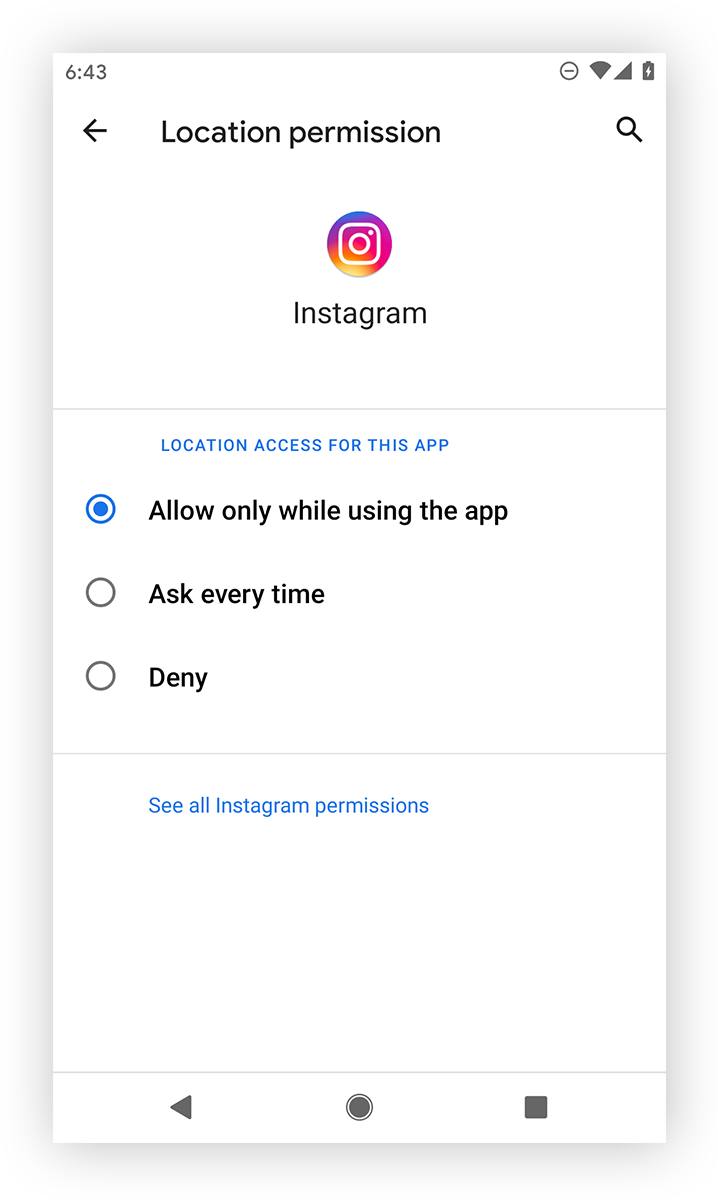Detailed Caption: 

A mobile screenshot displays the settings page of the Instagram app on a phone with a white background. At the top of the screen, the left-hand corner shows the time, "6:43." On the top right, there is an arrow pointing left, followed by the words "Location and permissions" and an icon of a magnifying glass. 

Beneath this top bar, a circular Instagram logo appears, resembling a camera. Below the logo, it reads "Instagram." A horizontal line separates this section from the settings options.

Highlighted in blue text, there is a title that says "Location access for the app." Underneath this, three options with circular radio buttons present different location settings. The first option, "Allow only while using the app," is selected, indicated by a blue-filled circle. The other two options, "Ask every time" and "Deny," are shown with empty circles, meaning they are not selected. 

Further down, another line of blue text reads "See all Instagram permissions." At the bottom of the screen, there is a navigation bar with an arrow pointing to the left, a circle, and a square. This image captures the entire settings page precisely as described.